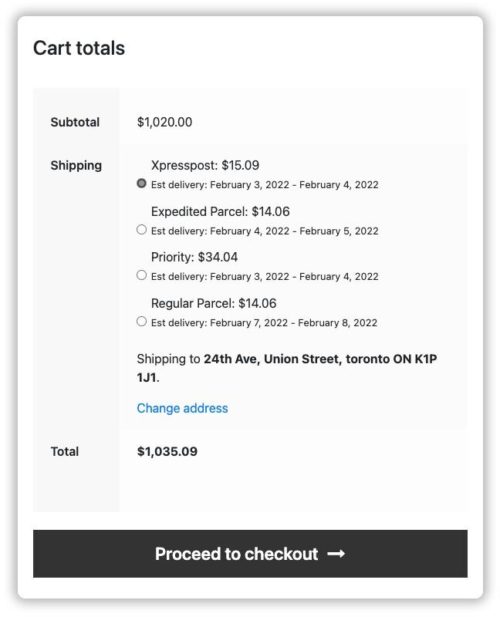The image depicts a cell phone screen showcasing the cart totals for an online purchase. At the top left corner, it prominently displays "Cart Totals." The subtotal for the items in the cart is listed as $1,020.00. Below this, the section labeled "Shipping" details four different shipping options along with their respective costs and estimated delivery dates.

1. **Express Post**: Priced at $15.09 with the selection circle filled in, indicating it is the chosen option. The estimated delivery dates are February 3, 2022 through February 4, 2022.
  
2. **Expedited Parcel**: Costing $14.06, this option has a blank selection circle and features estimated delivery dates from February 4, 2022 to February 5, 2022.
  
3. **Priority**: This more expensive option is priced at $34.04 with an unmarked selection circle. The estimated delivery dates are February 3, 2022 through February 4, 2022.
  
4. **Regular Parcel**: The least expensive at $14.06, this option also has an unmarked circle with delivery dates ranging from February 7, 2022 to February 8, 2022.

The shipping address is listed as 24th Avenue, Union Street, Toronto, Ontario, K1P1J1, with an option to change the address. The total cost for the purchase, including shipping, is $1,035.09. At the bottom of the screen, there is a prominent black button labeled "Proceed to Checkout."